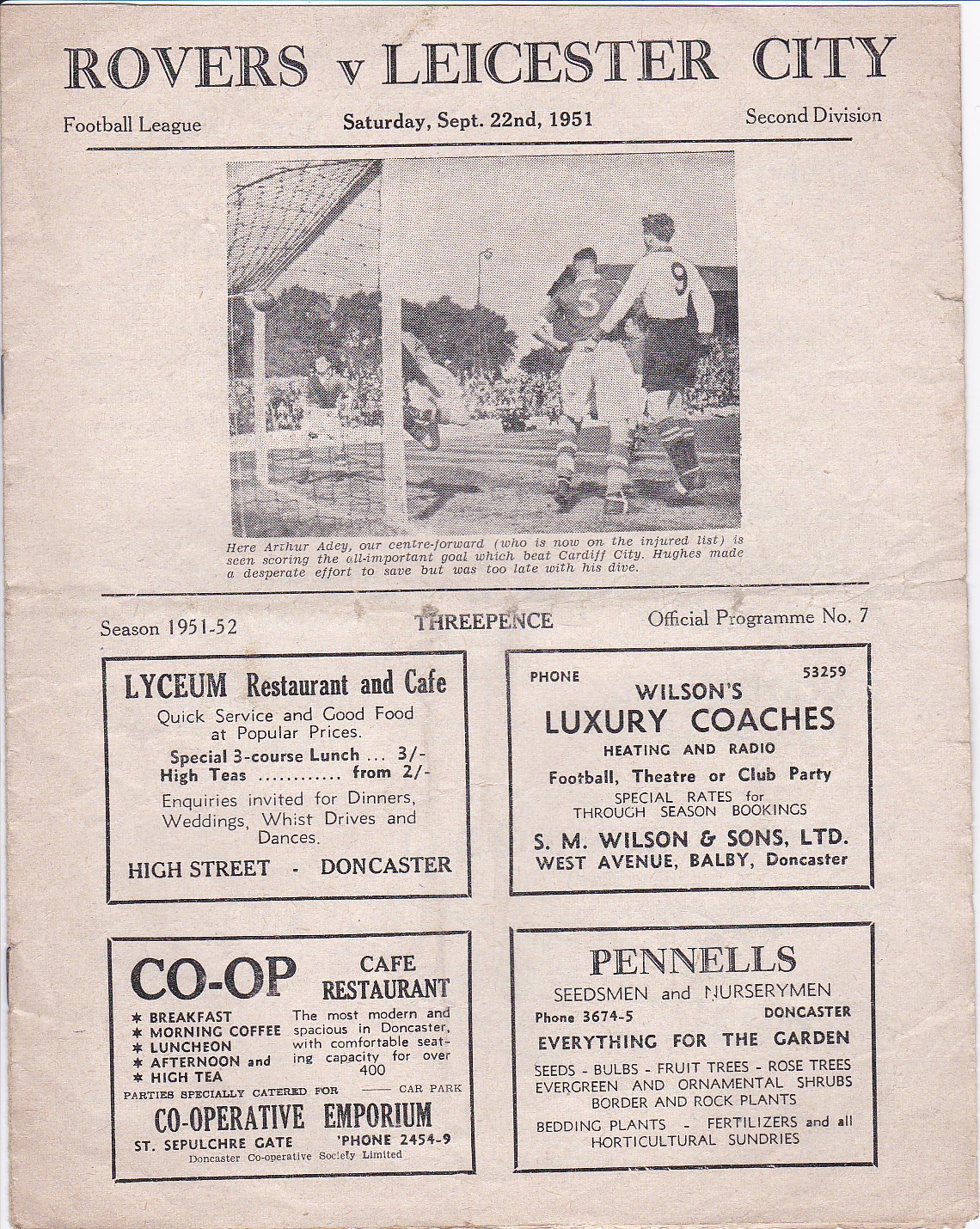The image showcases an old program page for a soccer match between the Rovers and Leicester City Football League, dated Saturday, September 22, 1951. The paper, which has yellowed over time, features black lettering set against a tannish background. At the top, it reads "Rovers v. Leicester City, Second Division," detailing the season as "1951-52," priced at three pence, and marked as the "official program number seven." Beneath the title, there is a small, black-and-white newsprint photograph of a soccer game, capturing two players near the goal line, one wearing a jersey with the number nine and the other with the number five. Below the image, various text blocks are laid out, followed by a series of four bordered advertisements typical of the era, promoting Lyceum Restaurant & Cafe, Co-op Cafe Restaurant, Wilson's Luxury Coaches, and Pennell's Seedsmen and Nurserymen.